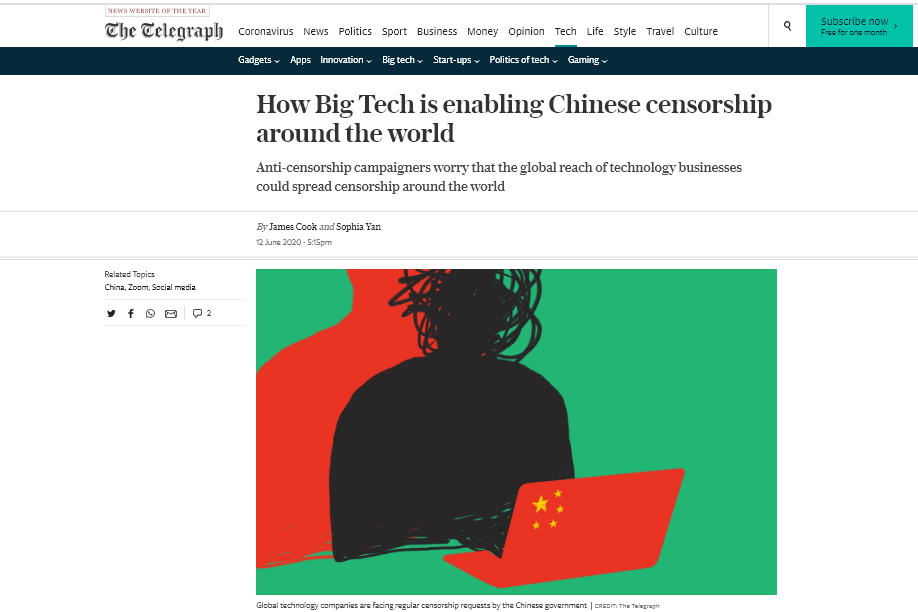A detailed screenshot of The Telegraph news website, captioned as "News Website of the Year" in the top left. The website's name, rendered in an old-timey calligraphy font, captures attention at the center top. The primary navigation menu displayed at the top includes categories such as Coronavirus, News, Politics, Sport, Business, Money, Opinion, Tech, Life, Style, Travel, and Culture, with a search icon and a green "Subscribe Now, free for one month" button located on the top right.

The Tech section is currently selected, highlighted by subheadings in white font on a dark background, offering options like Gadgets, Apps, Innovation, Big Tech, Startups, Politics, Tech, and Gaming.

The headline of the featured article reads: "How Big Tech is Enabling Chinese Censorship Around the World." The subheading elaborates, "Anti-Censorship Campaigners Worry that the Global Reach of Technology Businesses Could Spread Censorship Around the World," authored by James Cook and Sophia Yan, dated 12 June 2020, 5:15 p.m. 

On the left, a sidebar lists "Related Topics" which include China, Zoom, and Social Media, accompanied by social media sharing icons for Twitter, Facebook, WhatsApp, and email, along with a comments icon indicating two comments.

The main image for the article shows a silhouette of a person with a scribbled-out head, bathed in a red shadow, staring at a red laptop adorned with yellow stars reminiscent of the Chinese flag. The background is green. Below the image, a caption reads: “Global Technology Companies are Facing Regular Censorship Requests by the Chinese Government. Credit The Telegraph.”